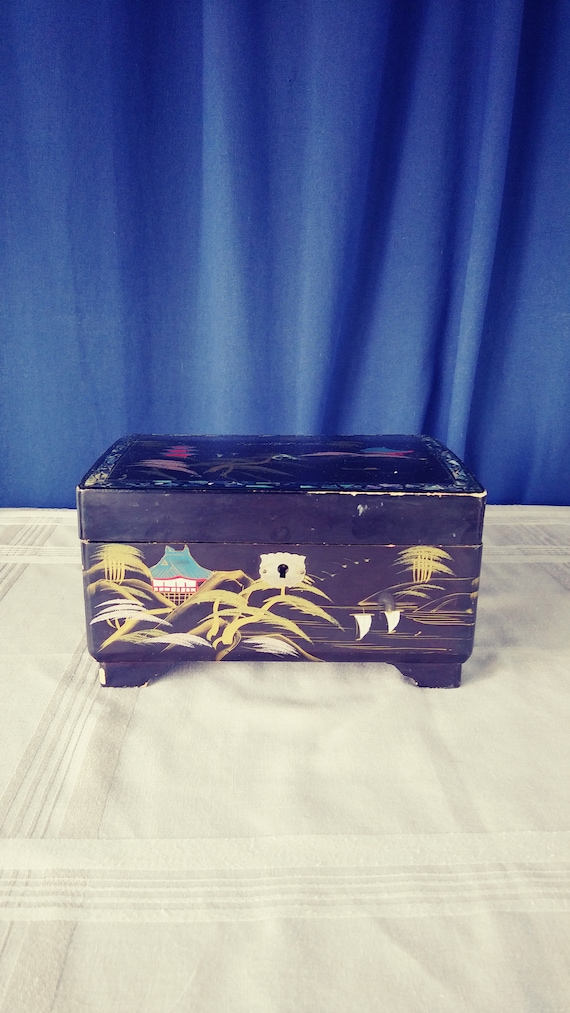The photo showcases a dark brown wooden chest, prominently featuring a keyhole in the middle of its front surface, suggesting it is a lock box. The chest is adorned with yellow paint streaks, possibly forming a design that might depict trees and a home. The chest rests on a light beige-colored cloth with a subtle pattern of cross marks. In the background, a blue curtain with numerous folds provides a contrasting backdrop. The image is well-lit and clear, offering a detailed view of the chest and its surroundings.